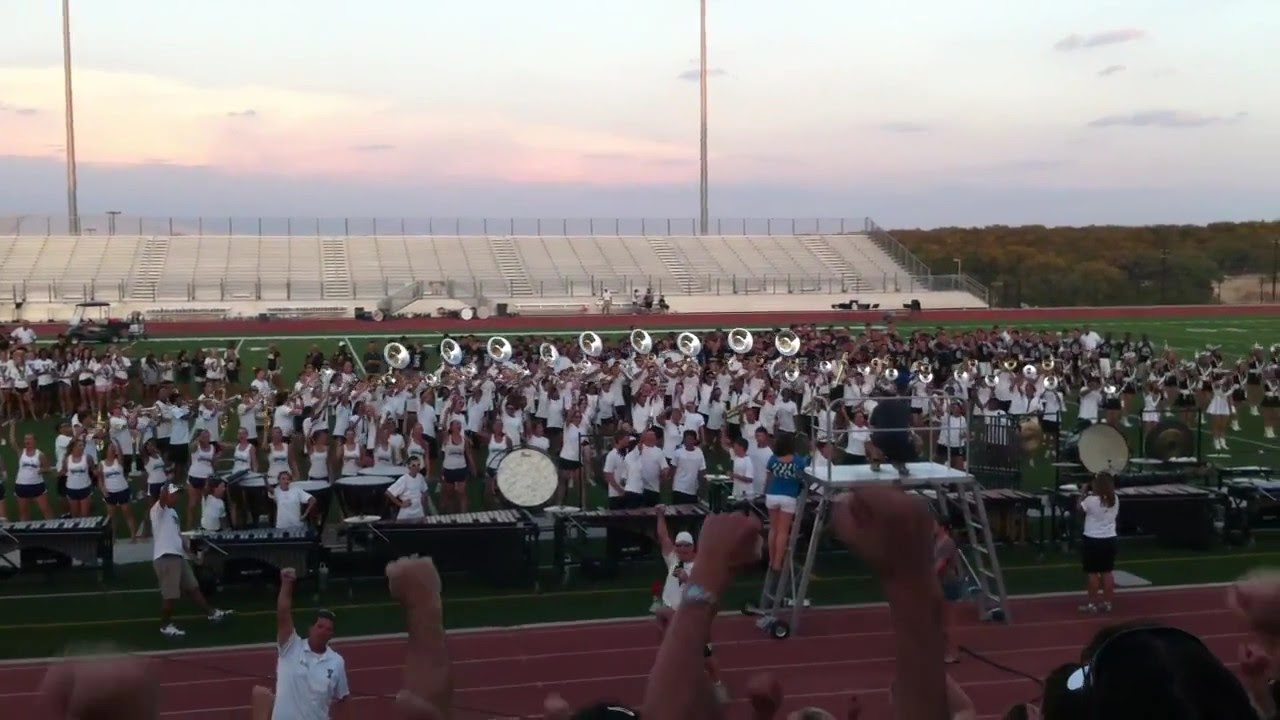This high-resolution photograph captures a serene, almost-sunset scene inside a football stadium featuring an impressive high school or college marching band. Arranged from left to right across the width of the field, the band members are uniformly dressed in white tops paired with dark pants. A striking feature is their silver trumpets and horns, the latter especially prominent in the middle of the formation. In the foreground, a man in a white shirt is seen waving to the photographer, framing the scene with a personal touch. 

Separating the band from the viewers is a track, maroon in color, and a fence along which various spectators stand, some with fists raised, seemingly in a cheer. The stadium's stands, visible in the background, are notably empty, adding a sense of spaciousness to the scene. Enhancing the composition are two poles behind the stands and distant trees, silhouetted against a light blue sky tinged with orange clouds, capturing the beauty of dusk. The image evokes a quiet, anticipatory mood before a performance, emphasizing the band's readiness and the audience's supportive engagement.